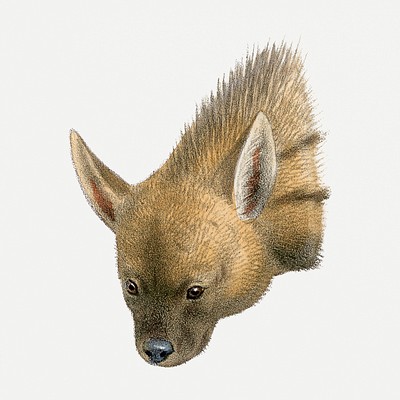The image is a detailed pen and ink drawing of an unidentified animal, focusing on its head and neck against a plain background. The animal has brown, spiky fur with two prominent, pointy ears that add depth to its face. Its facial features, including its black, beady eyes and a cute, oblong black nose, are reminiscent of a dog's or a bat's. The animal's tan fur is darker around its mouth and eyes, suggesting shades and texture similar to a hyena's. The fur on its neck has two brown stripes ascending towards the ears, giving it a striped appearance, despite the stripes being partially out of the frame. The ears are large and cone-shaped, with detailed shading to accentuate their form. The overall appearance suggests the animal might be an ancient or mythical species, brought to life through a pen and ink illustration, possibly enhanced with colored pencil or watercolor techniques, giving it rich texture and depth.